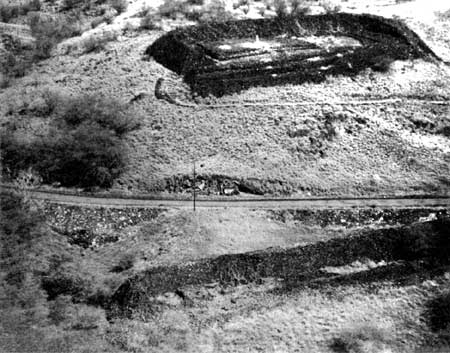This grainy, black-and-white photograph focuses on a landscape from a bird's eye view, presumably taken in the early 1900s, possibly from a helicopter. Dominating the scene is a road that cuts across the image horizontally, extending from the middle left edge to the middle right edge, passing through the lower half of the portrayed hill. To the left of the center, near this road, stands a lone power line pole.

The terrain is sparsely vegetated with bushes and trees scattered across the landscape. The photograph captures a rough yet distinctive feature at the top of the hill—a dark oblong mound of dirt, reminiscent of a fortified structure or possibly a mining site. This earthen formation has high, sloping walls resembling a stadium without stands or spectators. The inside of this mound descends into a flat, lower center, creating an impression of a hollow dugout bordered by elevated sides. A faint pathway can be discerned winding up to the left side of this mound, encircling the structure and heading off towards the right side of the image. The overall impression is of a somewhat otherworldly or model-like landscape punctuated by notable topographical features.